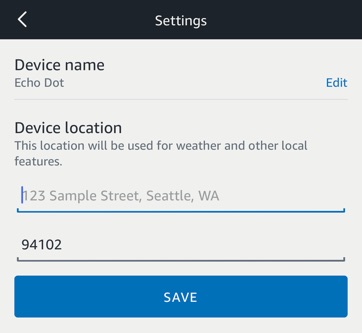This is an image of a settings page. The page has a vertical orientation, being slightly taller than it is wide. At the very top, there is a black border running horizontally across the width of the page. Within this border, there is a small, white arrow pointing to the left, and centered in the middle in white text is the word "Settings."

The remainder of the page features a gray background. Just below the black border, the words "Device Name" appear in black text. Beneath this, also in black text, is "Echo Dot." Aligned to the far right of the page, in blue text, is the word "Edit."

Further down, the words "Device Location" are displayed in black text. Below this, in slightly smaller black text, is a note saying, "This location will be used for weather and other local features." Following this, there is an address: "123 Sample Street, Seattle, Washington," underlined by a blue line. Below this address is the ZIP code "94102," also in black text. This section is separated from the lower part of the page by a dark gray line.

At the very bottom of the page is a large, medium blue rectangular button, which spans almost the full width of the page. Centered within this button, in all capital letters and white text, is the word "SAVE."